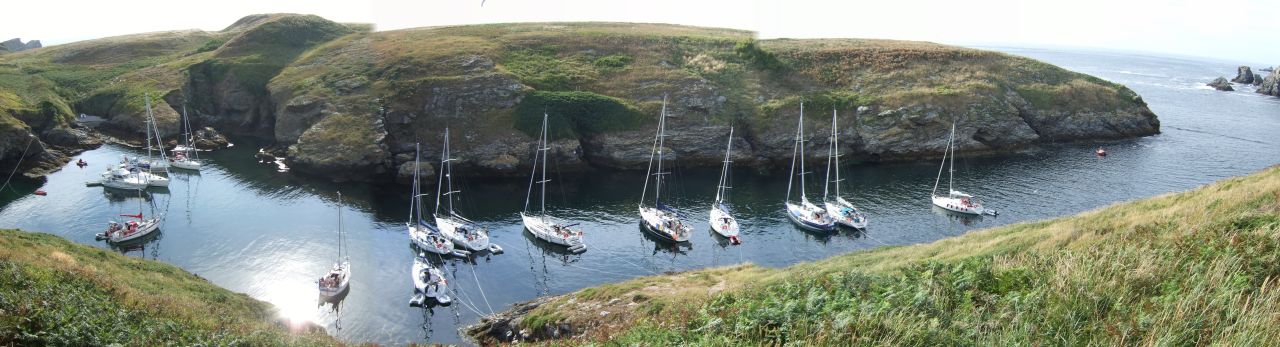This panoramic aerial photo captures a verdant, rocky inlet dotted with at least a dozen white sailboats, their masts standing tall but noticeably devoid of sails. The scene is framed by lush, grassy cliffs that form a natural boundary around the water, resembling a short, fat hockey stick in shape. The bright, possibly overcast sky provides a high-contrast backdrop, making it difficult to discern any cloud patterns. The cliffs, covered in green grass and moss, descend steeply to this serene water channel, which opens up to the ocean on the far right. The boats appear small and closely positioned, floating placidly on the water, creating a picturesque and tranquil marine landscape with a unique geometric perspective.